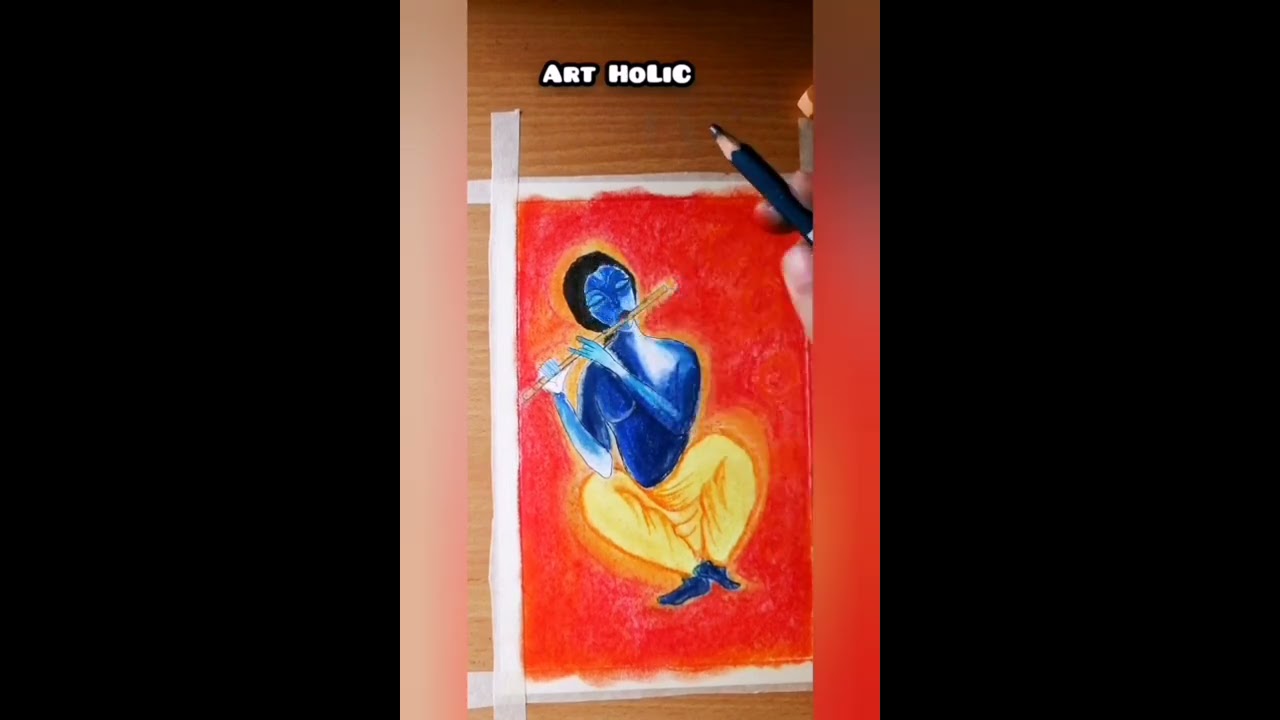In this detailed image, we see a vibrant drawing positioned at the center of a plain black background, held down by white masking tape on a wooden table. The top of the image prominently features the text "ART HOLIC" in bold, white, bubbly capital letters. The artwork depicts a blue-skinned character with dark hair, wearing flowy yellow pants and blue feet, sitting in a squatting posture against a red background. The character, resembling an Avatar-like figure, holds a flute with both hands. The overall style suggests a blend of painting and colored pencil or chalk drawing, with the character's face displaying a Picasso-esque shape. Visible in the top right corner is a hand with a blue pencil, adding to the art, suggesting an active creation process. The composition is surrounded by black borders, with a small portion of the creator's hand visible, adding a sense of immediacy and personal touch to the piece.